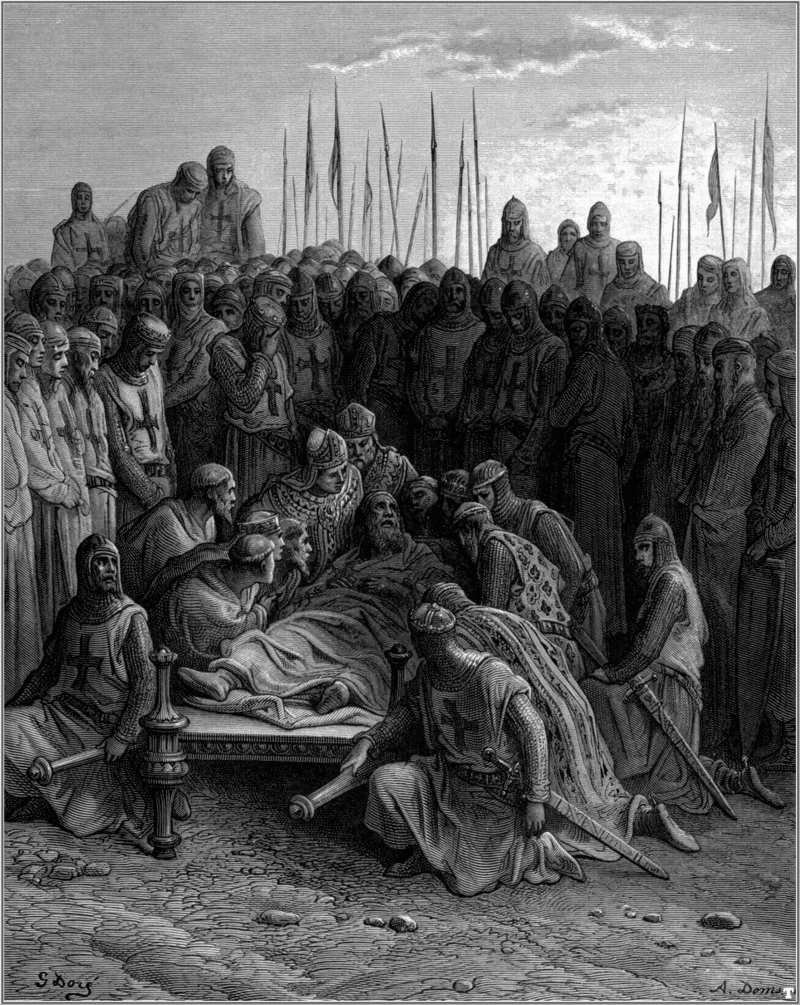This black-and-white image, which could be a painting or engraving, depicts a poignant scene from the time of the Crusades. At the center, a man, dressed in long robes, lies on a bed, clearly sick or dying, and gazes upward. Surrounding him are crusaders, recognizable by their historical attire adorned with crosses around their necks and on their chests, and armed with swords and spears. They display a mixture of postures—some kneel beside him, bending over in concern, while others stand or hover with solemn expressions, one even weeping with his head in his hands. In the backdrop, a multitude of crusaders, numbering between 20 and 30, can be seen, some standing elevated as if on a platform, all facing the central figure, adding depth to this scene. Flags and an overcast sky with varying shades of gray enhance the grim atmosphere. The image, marked with an 'S' and 'D-O-Y' on the bottom left, and 'A.D.' on the bottom right, evokes a scene of collective prayer or farewell during a significant historical moment, rendered entirely in black, white, and shades of gray.